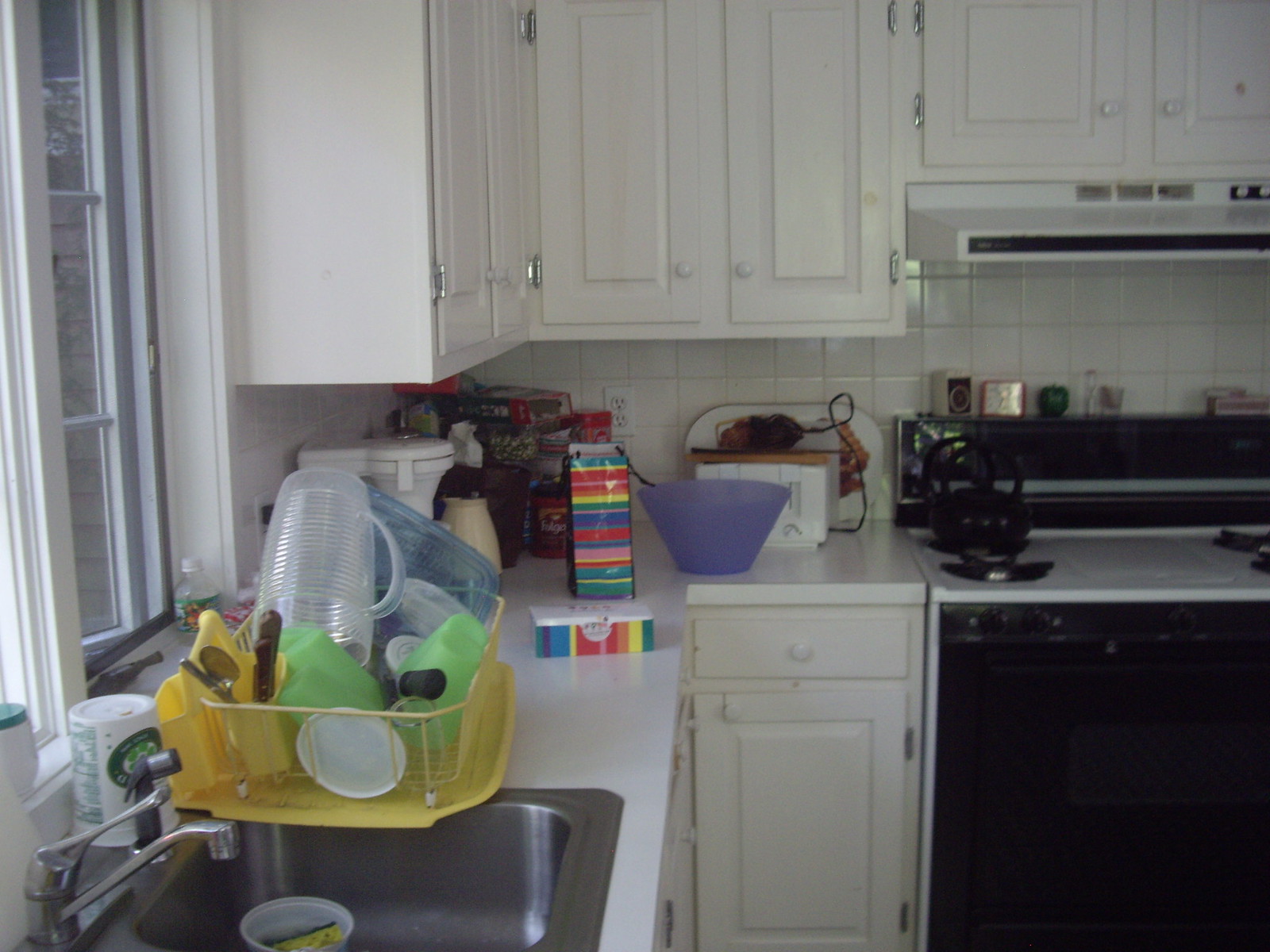The image captures a bustling small apartment kitchen, marked by its compact and utilitarian design. Central to the scene are white cabinets that span both the upper and lower portions of the kitchen, framing the space symmetrically. To the left of the cabinets, an open window invites light into the room. In the bottom left corner, a sink sits beneath the window, adorned with a pile of freshly washed dishes resting in a drip-dry container, signaling the recent conclusion of dishwashing. A cup holding a sponge lies at the bottom of the sink, reinforcing the notion of ongoing kitchen chores.

Moving up along the left side, partially hidden behind the dish rack, an old-school, white coffee maker quietly occupies its space. Adjacent to it, a cluttered mix of bottles and containers adds to the kitchen's lived-in feel, though their specific nature remains indistinct. The white backsplash behind these items matches the white cabinets, creating a cohesive visual theme.

Dominating the center of the image is a white toaster oven, which stands out against its surroundings yet is partially blocked by a purple bowl. To the far right, the kitchen range comes into view, predominantly white with a black oven door. On the back left burner, a black teapot blends with the stove’s surface, adding a touch of everyday functionality to the scene.